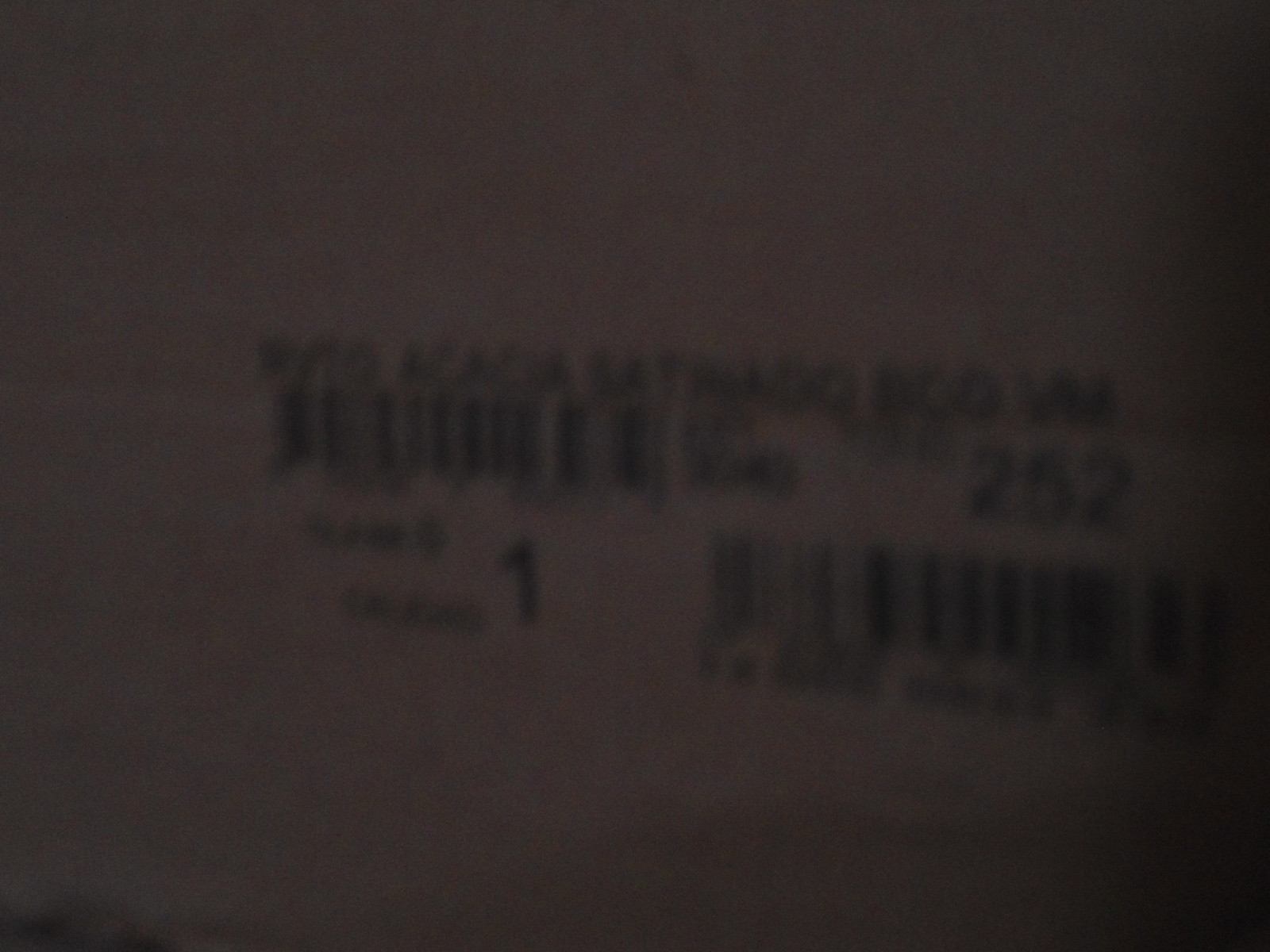The image depicts a dimly lit, blurry label on a box, possibly taken in a dark room or with intentional low lighting. The label appears predominantly in dark gray or possibly dark brown hues, with black text and numbers, making it difficult to read clearly. At the top of the label, there's an unreadable sequence of letters, followed by a prominent barcode beneath it. Below the barcode, there are more letters, with the number "1" visible in the center. On the right side, there's another set of letters and numbers, including a large, black "252." Further down, another barcode is visible, and at the bottom right, there's a mix of additional numbers and letters. The focus is entirely on this label, and the rest of the image does not provide any context or background details.